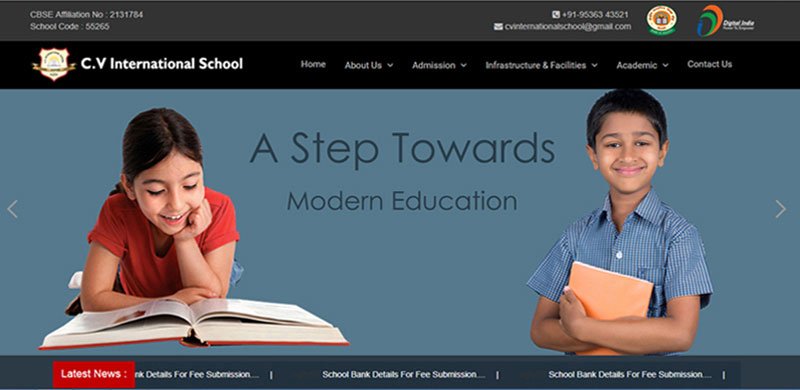This is a screenshot of a website with a dark and slightly blurry background. At the top left corner, on a light gray bar, there is text that reads "CBSE Affiliation No. 2131754". Beneath it, there is a smaller text that says "School Code: 56265". On the top right corner, a phone icon is followed by the number "+91 9536343521". Just below this, there's an envelope icon with an email address: "cvinternationalschool@gmail.com". 

To the right, there is a light-colored logo next to a tri-colored logo in blue, green, and red, forming a 'D' shape with the text "Deep India" written underneath it. Below this, on the left side, a yellow shield with white text stating "CV International School" can be seen.

The website menu is positioned below these elements, listing the options: Home, About, Mission, Infrastructure & Facilities, Academics, and Contact Us.

In the middle of the screen, there is an image of a girl with brown hair looking down at a book and smiling while lying on the ground. To the right of her, a boy in a blue shirt holds a book and smiles directly at the camera. Arrows pointing left and right are located next to the boy’s image. 

A tagline beneath these images reads "A Step Towards Modern Education".

Below this section, there is a gray bar with a red box labeled "Latest News". Inside the gray bar, the following announcements are made: "Details for Fee Submission" is repeated three times in the center and on the right side.

Overall, the displayed website seems to emphasize educational information, contact details, and current announcements for fee submissions.